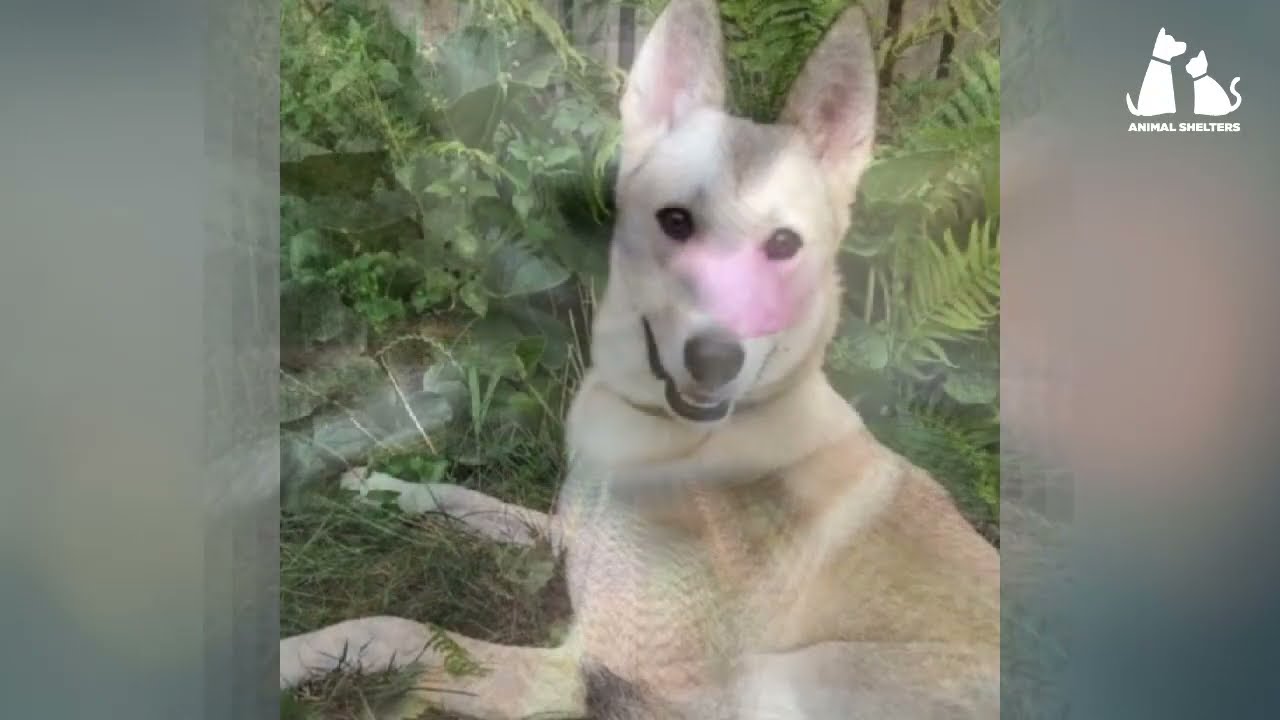This photograph features a slim, white and brown dog with tall, perked ears and a slightly open mouth, giving the impression of a smile. The dog, which resembles a hunting breed, is captured sitting in lush, green grass with its front paws extended forward. Its intelligent eyes, black nose, and attentive posture suggest alertness and curiosity. The background showcases green foliage including vines, palm fronds, and ferns, adding to the natural outdoor setting. The image appears slightly altered with added pink hues over the nose and eyes, and it is noted that the photograph is somewhat blurry. Vertical grey strips frame the sides, and the top right corner features a logo with the outline of a dog and a cat, and the text "Animal Shelters," indicating a connection to pet adoption or animal care.